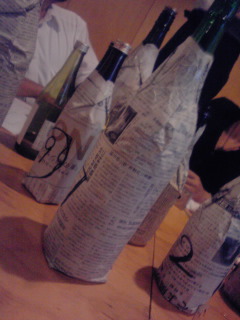In this color photograph taken indoors at an angle, several dark green bottles with dark screw-on caps are tightly wrapped in newspaper and arranged on an orange, tiled wooden table. The newspaper is illegible, but some bottles bear numbers written in black marker, such as a number 9 encircled and a number 2. In the background, an unwrapped clear bottle with a silver cap stands out, while partially visible are two people: one wearing a white shirt and another in a black shirt. The lighting is poor, casting strong shadows towards the left, and creating a dim, moody atmosphere. A grey triangle appears in the upper left-hand corner, and the image is tilted to the right, emphasizing the skewed perspective.